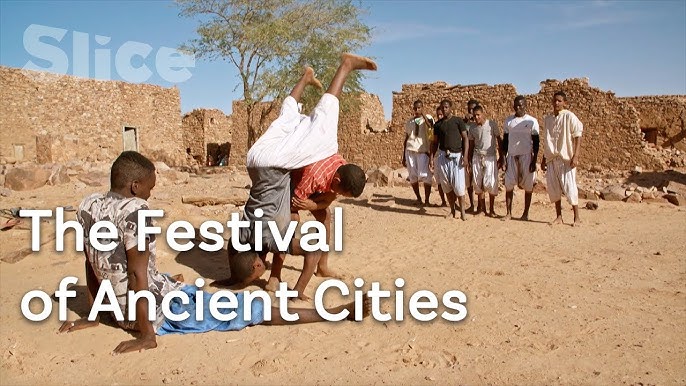In this vibrant image, set against a backdrop of a vast blue sky with wispy white streaks, a lively outdoor scene unfolds. The upper left corner subtly features the white text "slice," and in the bottom left, it reads "The Festival of Ancient Cities" in a similar font. Dominating the foreground, two children engage in playful stunts on a light brown, sandy ground. One child, wearing white pants and a gray shirt, is balanced upside down on his hands, supported by another child in a red-striped shirt with short hair. Nearby, a male child sits on the ground with his hands planted behind him, legs stretched out, dressed in blue shorts, observing the energetic play.

In the middle ground, a group of men, some in black shirts and others in white, stand attentively, watching the children. This group includes several black men, highlighting a diverse community spirit. Behind them, ancient stone buildings, some appearing well-preserved and others in decay, form a rugged skyline. These tan structures, evocative of a historical era, contrast with the solitary, slender tree on the left, its thin green leaves and branches swaying lightly in the warm, temperate breeze. The overall scene encapsulates a moment of communal joy and cultural celebration under a radiant sun.